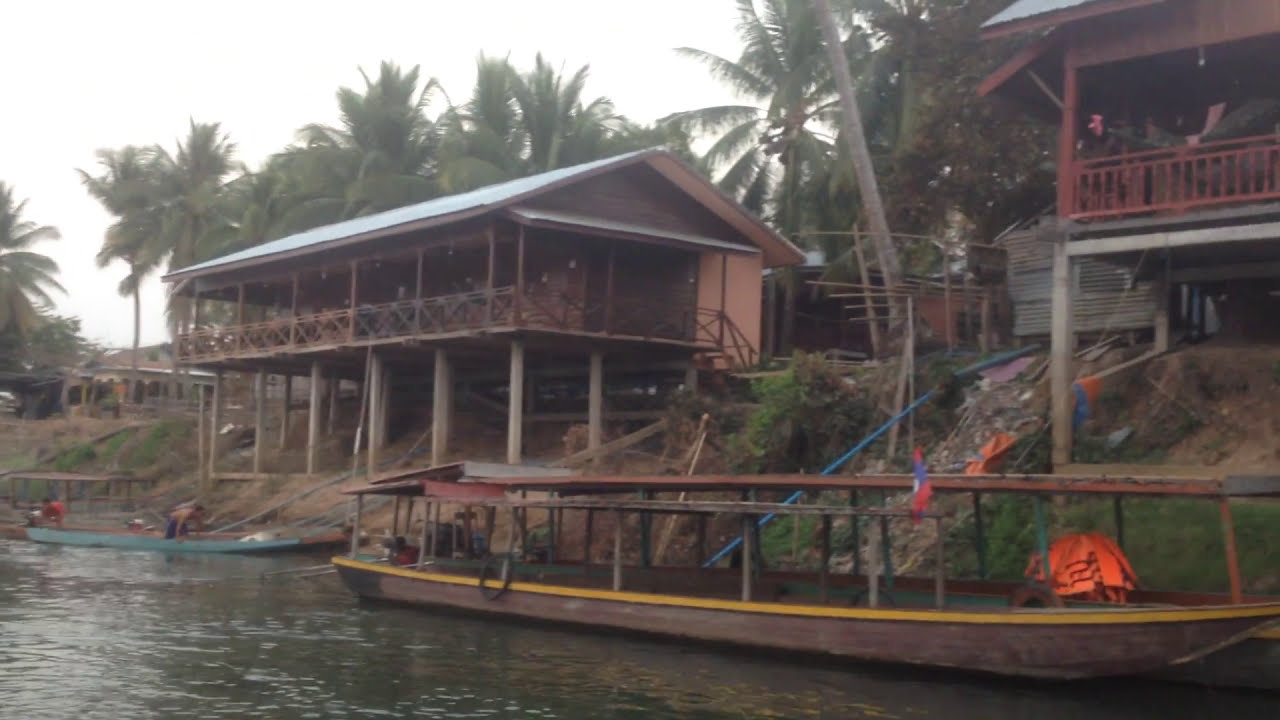The image depicts a tropical riverbank scene with a somewhat overcast yet bright sky. In the foreground, there is a long, wooden boat adorned with a white stripe and equipped with orange life jackets towards its front. The boat, which can accommodate approximately eight people, has a few individuals around it; one man is bending over inside, while another stands at its end. Adjacent to this boat is another smaller motorboat with a couple more people. 

The riverbank itself slopes upward into a hill where several buildings on stilts are situated, likely to protect them from rising tides. These structures have two stories, with the first level elevated on stilts and connected by red railings on the second floors. The area around these buildings is cluttered with loose posts and boards. In the background, an abundance of palm trees suggests a lush, tropical environment. Additionally, there appears to be a blue, red, and white flag on one of the boats, though it is not the American flag. Overall, the image, although somewhat fuzzy and grayed out, captures a serene and somewhat busy riverbank scene in a tropical setting.